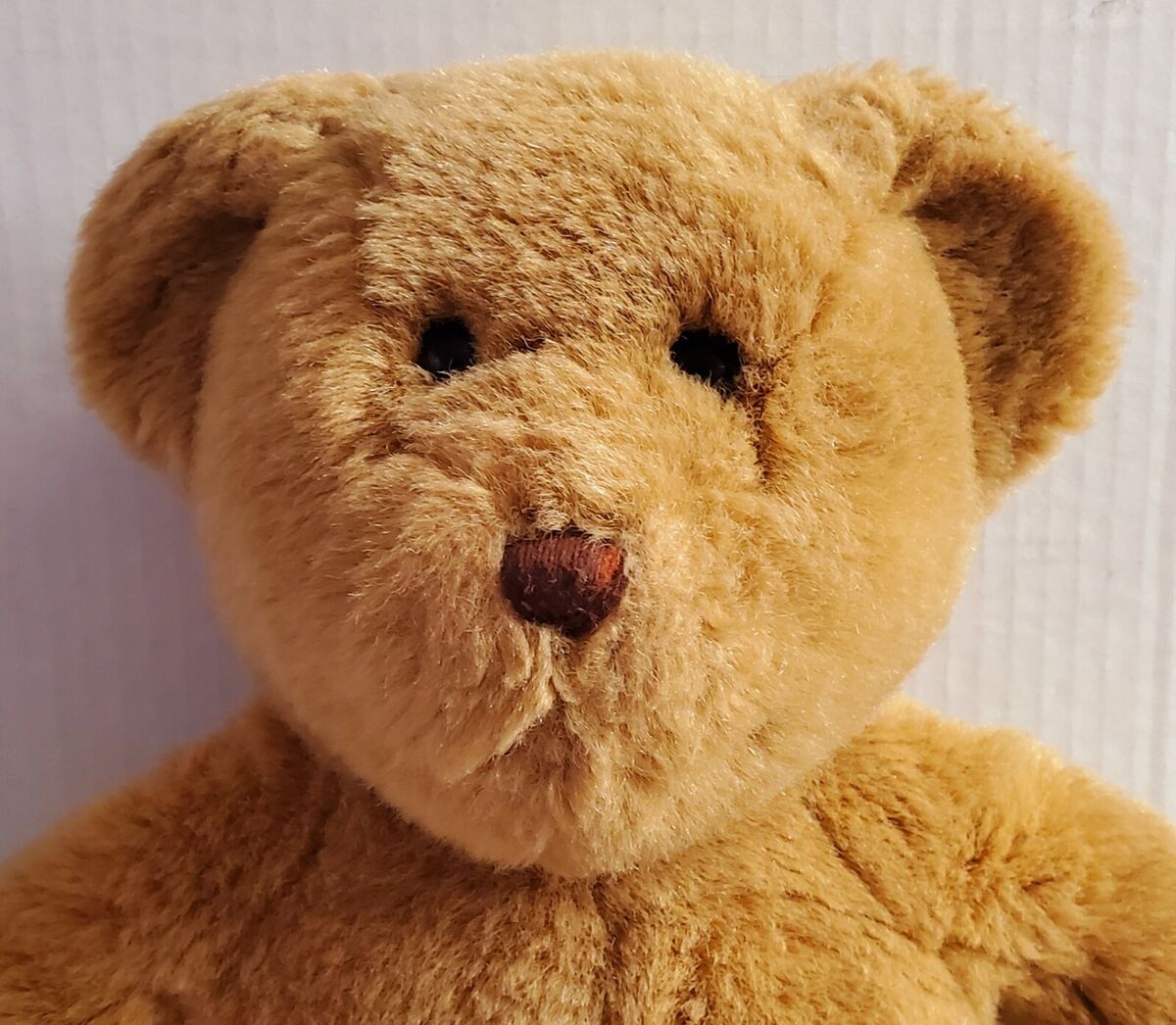The image is a full-color, square photograph taken indoors with a subject that is prominently a light brown teddy bear, occupying the majority of the space. The background is a vertically corrugated, gray-toned surface, giving an industrial texture to the staged setting. The teddy bear, positioned centrally and facing the viewer, is depicted from the top of its rounded ears down to just below its shoulders. It has small round black eyes that sit above a stitched brown nose, slightly reddish in hue, with no visible mouth or clothing, suggesting a simplistic and classic design. The furry head of the bear is triangular at the bottom and rounded across the top, seamlessly extending into its shoulders, which taper down towards the bottom corners of the image. The lighting leaves ambiguity, making it unclear whether it is natural or artificial, but it highlights the bear's soft texture and neutral expression in a detailed representation.